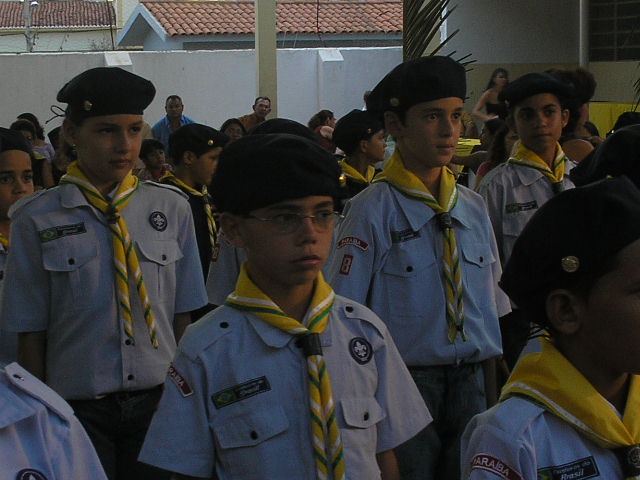The photograph captures a gathering of young boys in Boy Scout uniforms, standing at attention, possibly during a ceremony or event. They are uniformly dressed in light blue shirts adorned with emblems and name tags, featuring two front pockets. Around their necks, they wear yellow neckerchiefs with red, green, and white stripes, tied neatly. Each boy also wears a dark beret with a pin. In the background, partially visible under a dim daytime lighting, are several white-walled buildings topped with brown Spanish tile roofs, suggesting an outdoor setting with an architectural flair not typical of America. There are adults—men and women—clustered in the background, likely parents or family members, adding to the communal feel of the scene. No specific identifying information, such as names, date, or location, is present in the image.